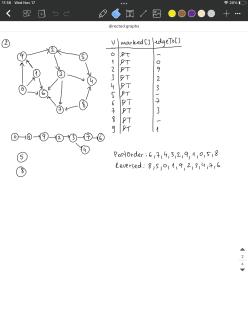The image is a screenshot of a computer program used for capturing handwritten notes or annotations. The interface at the top of the screen displays various UI elements including color selection options, tool selection icons, and other standard software functions. Below this interface, the main handwritten segment of the image begins.

On the right side of the handwritten area, there is a grid with three columns. The grid is titled "V" on the left and lists numbers from 0 through 9 vertically. The middle column is labeled "Marked" and features letters "P" that have been struck through with a "T" in each row. The right column has a title that is not clearly legible, with some rows containing values while others are empty.

On the left side of the handwritten notes, there is a diagram that connects different numbers, followed by another distinct diagram below it. Finally, there is a cross-check list situated beneath the previously mentioned grid, containing various additional details and annotations.